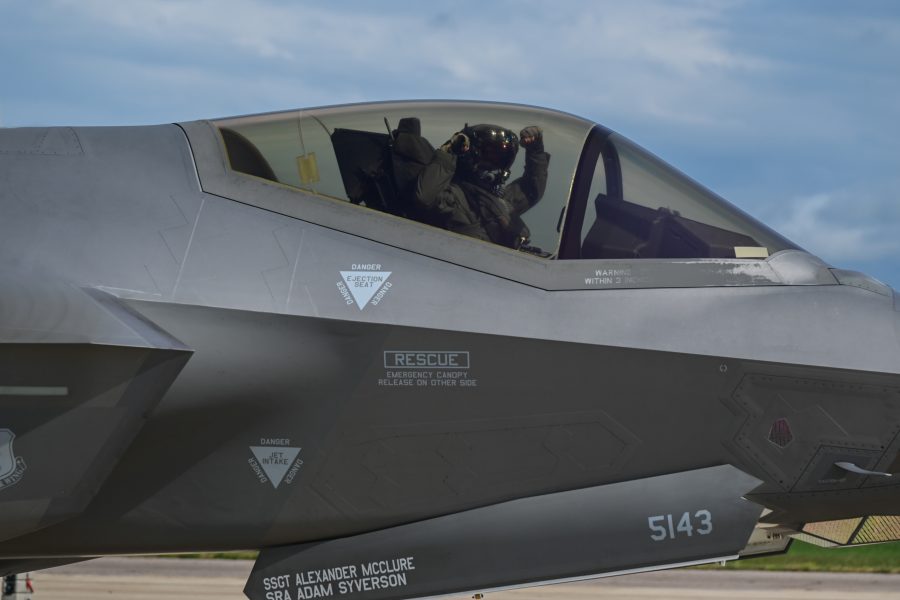The image depicts a dark gray fighter jet with clear text on its side, featuring personnel names "Senior Sergeant Alexander McClure," partially cut off text likely reading "SRA Adam Siverson," and the aircraft identifier "5143." Prominently displayed near the top of the jet are safety instructions, including "Rescue Emergency Canopy Release on other side" and various warning labels such as "danger" and "ejection seat." The jet's cockpit is covered by a slightly tinted, see-through canopy. Inside the cockpit, a man is visible, dressed in a pilot's uniform and helmet, his face obscured. His arms are lifted above his head, possibly adjusting his face mask or preparing for takeoff. The background reveals a clear blue sky with minimal clouds and gray concrete ground, suggesting the plane is on a runway or tarmac. The abundance of warning labels contributes to a perception of the aircraft's inherent dangers.